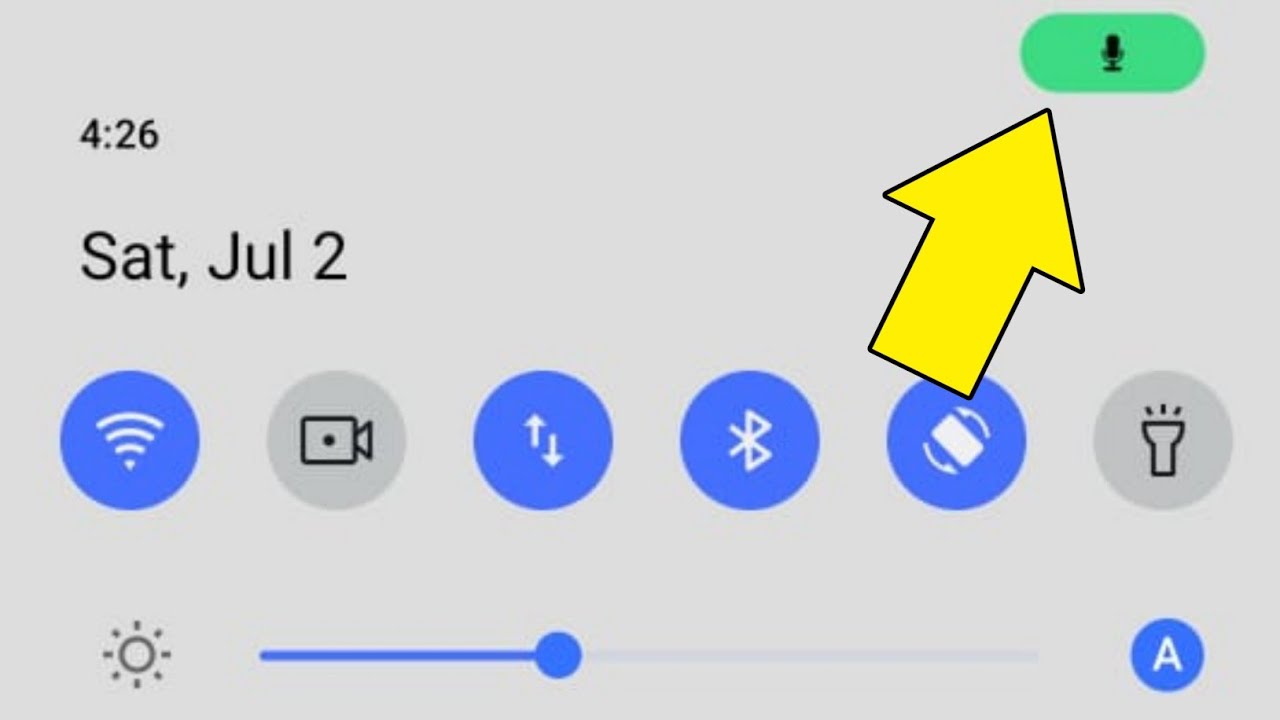In the image, there is a gray rectangular interface with a wealth of detailed symbols and text elements. On the far left side of the rectangle, the time "4:26" is displayed, though it's unclear whether this is a.m. or p.m. To the immediate right of the time, there is a solid green oval featuring a black microphone symbol at its center. Within the lower left portion of this green oval sits a prominent, bright yellow arrow bordered in black.

Moving to the right-hand side of the rectangular interface, there's text indicating the date "SAT, JUL 2" (Saturday, July 2nd) in uppercase letters. Below the date are several circles, each containing distinct symbols. The first circle is blue with a Wi-Fi signal icon. The second is gray and displays a black camera. The third is blue again, featuring a white arrow pointing upward and another pointing downward. The fourth blue circle is marked with an unfamiliar symbol resembling two white triangles with a circle at the center. The fifth blue circle, partially obscured by the yellow arrow, displays an icon with a rectangle and an arrow beneath it. Finally, the last gray circle shows a black flashlight icon.

At the bottom of the image, there is a gray sun symbol functioning as a brightness control slider. Part of the slider bar is blue, indicating adjustable light intensity, with a blue circle to show the current brightness level. Additionally, a blue circle containing a white letter "A" is positioned at the very end, possibly indicating an auto-brightness feature.

Overall, the image presents a complex user interface, depicting elements that suggest time, date, audio controls, connectivity status, and brightness settings.